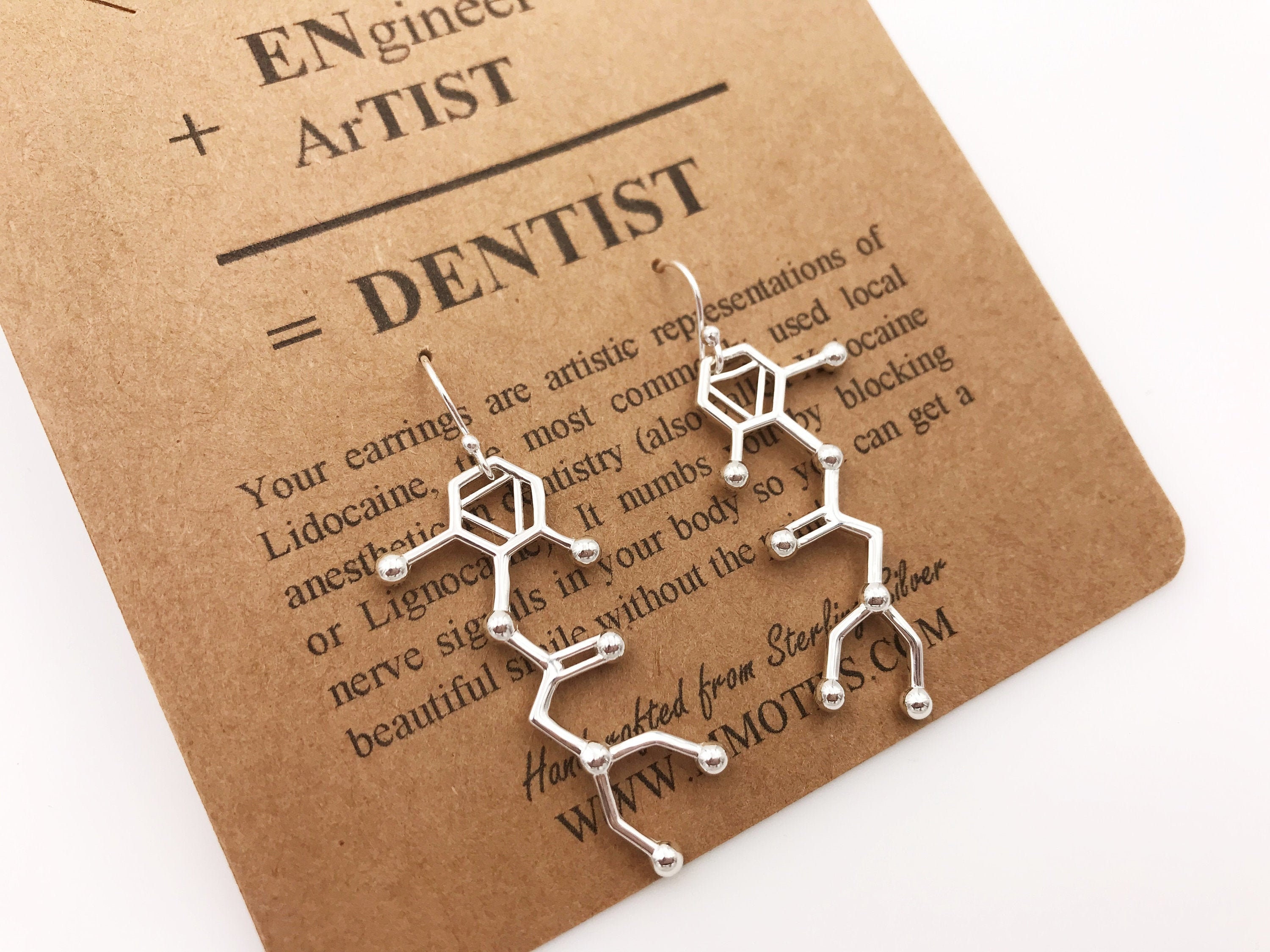This detailed color photograph, rectangular in shape, features a pair of sterling silver pierced earrings designed as artistic representations of the lidocaine molecule, commonly used as a local anesthetic in dentistry. The earrings, with intricate geometric shapes depicting hexagonal and elongated molecular structures, hang from a brown card set against a very light cream background. The top of the card reads "ENgineer + ARTIST = Dentist," with the capitalized 'EN' in Engineer and 'ARTIST' standing out. Some of the text is obscured, but it clearly mentions that the earrings symbolize lidocaine, numbing the body by blocking nerve signals to enable a pain-free, beautiful smile. The card also states that the earrings are handcrafted from sterling silver, with a partially visible web address, likely www.something.com.